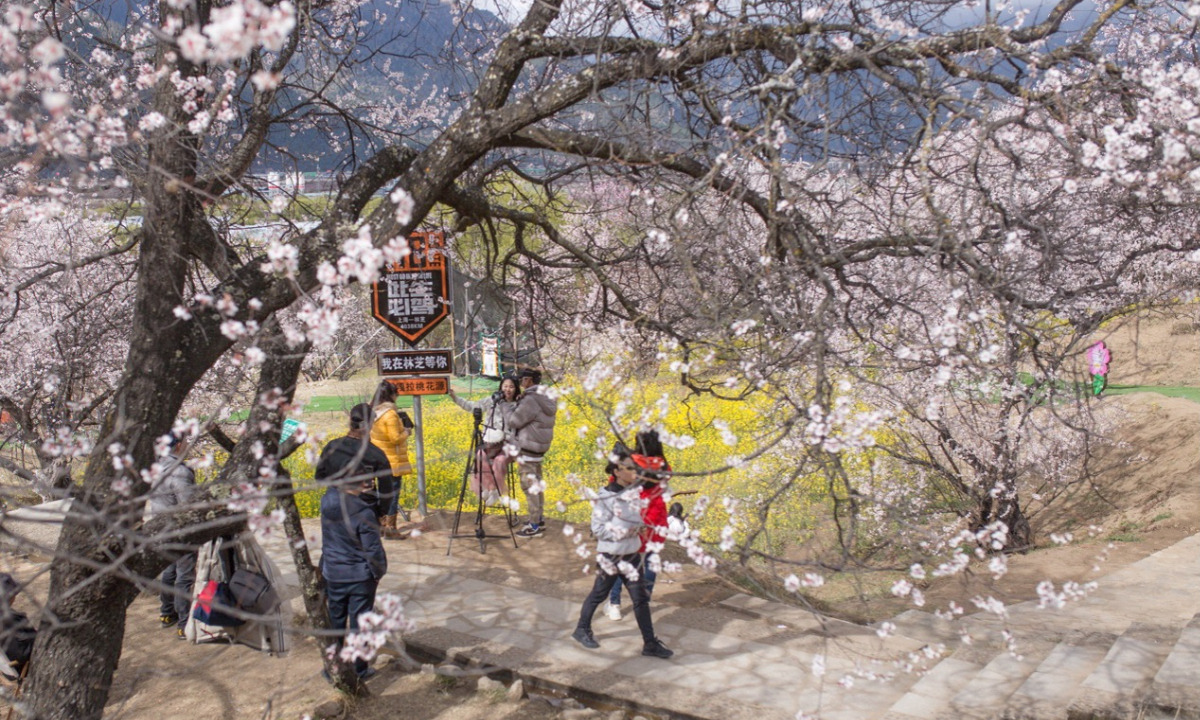The image depicts a picturesque scene in a Japanese park, likely during the Cherry Blossom Festival. Dominating the view is a tree adorned with plentiful light pink cherry blossoms, creating a breathtaking canopy. The scene is set along a light grey, whitish path where various people are promenading. Notably, a woman in a white coat is walking along the sidewalk, possibly carrying someone. In the backdrop, a couple stands close together, smiling, with a camera set up on a tripod aimed at them, suggesting they might be capturing a special moment like an engagement or wedding. They're situated near a series of signs: an orange sign with black and white letters, followed by another sign with white letters on a black background, and yet another orange sign with black lettering. Among the onlookers, a woman in a yellow coat and another in a pink coat add pops of color to the scene. The setting is vibrant, marked by contrasting elements of nature and human activity, amidst the gentle glow of blossoms and various visitors enjoying the celebration.